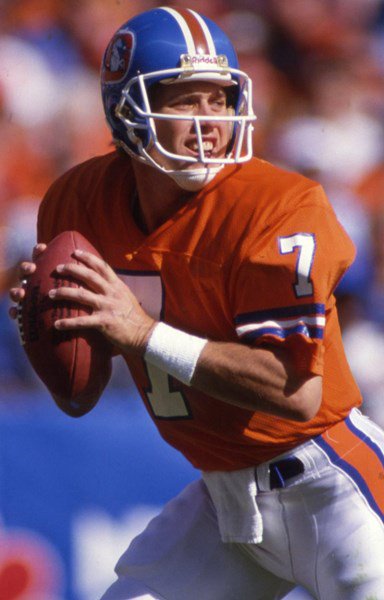This is a detailed photograph of a vintage quarterback, evident by his gear and uniform style. The focus is solely on the player against a blurred background. The quarterback, a Caucasian man with an open mouth revealing his teeth, is poised to throw the brown football he grips in both hands. He's dressed in a burnt-orange jersey with blue and white stripes on the sleeves, featuring a prominent white number 7 bordered in blue. His white pants have blue and orange stripes on the sides, secured with a black belt with a silver buckle, and a white towel tucked into the waistband. His blue helmet, adorned with a white stripe flanked by blue stripes down the center and equipped with a white metal face guard and a white cup chin guard, completes his retro ensemble.